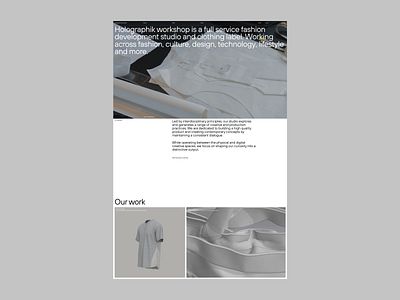The image appears to be a digital mockup of a portfolio-style webpage for a fashion company called "Holographic Workshop." Set against a light gray background, the vertical layout is divided into three distinct sections. The top section features a black-and-white photo of paper reams with fabric patterns and a bold, white, vertically left-aligned text that reads, "Holographic Workshop is a full-service fashion development studio and clothing label working across fashion, culture, design, technology, lifestyle, and more." 

Beneath this, a white section with black text likely acts as an introductory paragraph or further description, though the text is blurred and unreadable. In the lower part of the page, a bold subheading states "Our Work," flanked by two images: the left image showcases a detailed 3D rendering of a gray short-sleeve t-shirt against a matching gray background, while the right image presents an abstract, geometric bundle of white fabric. The minimalist color scheme, utilizing primarily gray, black, and white, complements the clean and modern aesthetic of the design.